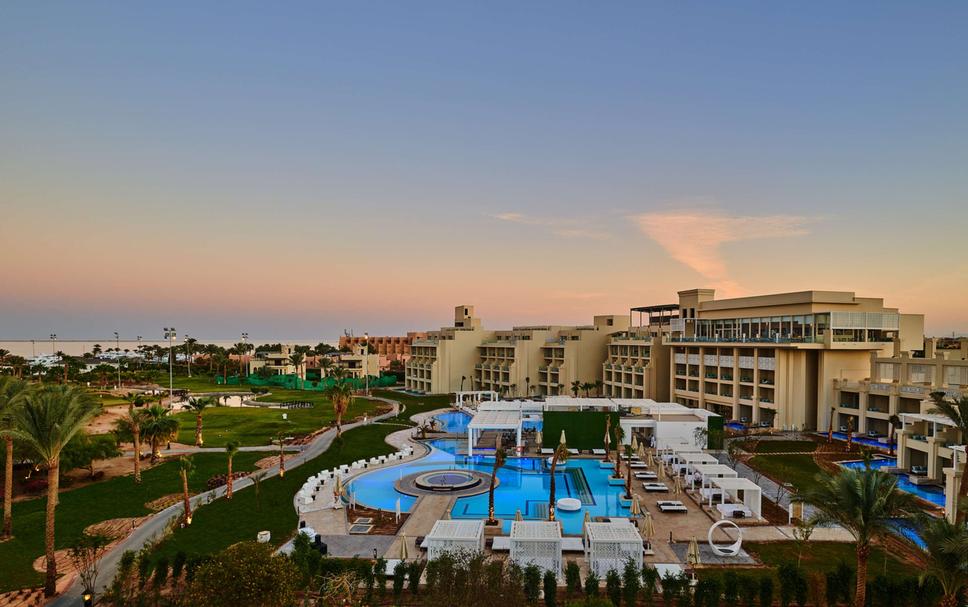The image captures an expansive resort setting transitioning into a peaceful sunset. Dominating the foreground is a very large, clear blue swimming pool that extends across the frame, punctuated by cabanas, lounge chairs, and a pool house. Multiple canopies and umbrellas offer shaded spots to relax, while neatly manicured lawns and various palm trees, both large and small, add greenery and tropical charm. A paved path flanked by palm trees meanders along the left side, leading the eye towards the horizon lined with several identical, imposing buildings resembling villas. In the distance to the far left, the ocean peeks into view, adding a serene backdrop to the lively scene. The sky above is a mesmerizing blend of pink, blue, and amber hues typical of a setting sun, streaked with wispy white clouds. The overall scene conveys a harmonious blend of natural beauty and luxurious architecture.